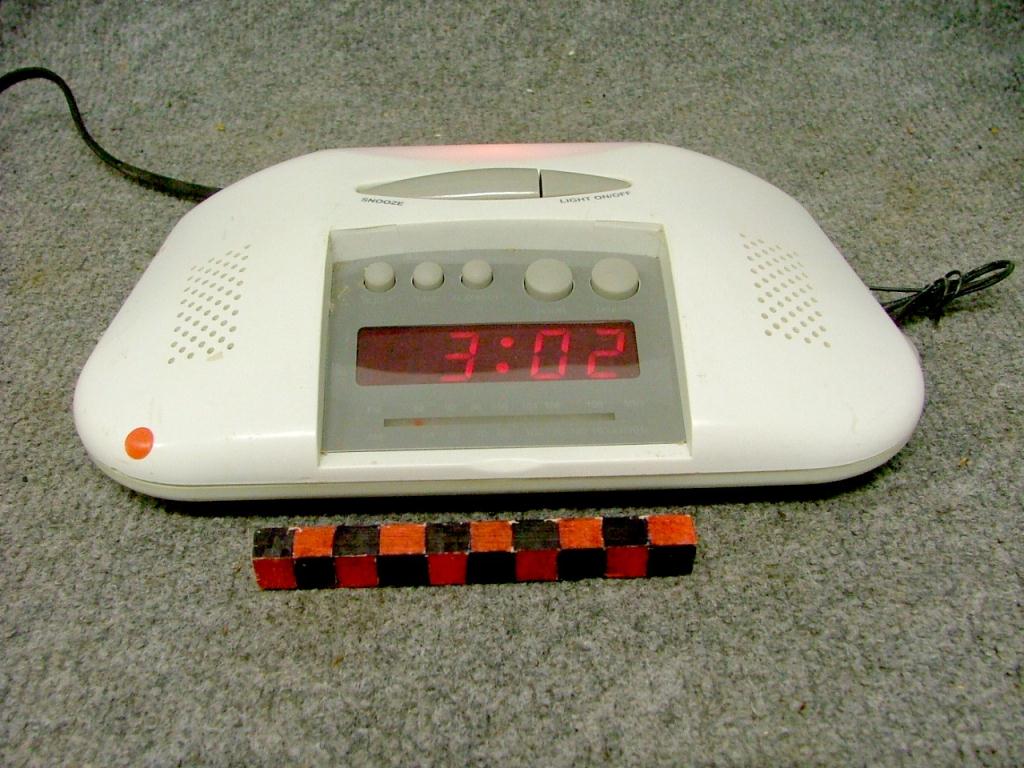The image features a white alarm clock placed on a coarse, gray carpet. The clock, positioned on the floor, prominently displays the time "3:02" in a red digital format at the center. Flanking the sides of the clock are built-in speakers. At the top of the clock, there are two buttons: a larger snooze button and a smaller button for toggling a light on and off. Additionally, three small buttons can be seen on the left side of the clock, while two larger buttons are situated on the right side. Extending from the top left corner of the clock, a power wire trails off out of the frame. On the right side of the image, a coiled antenna wire is visible. In the foreground, a small checkered stick-like object is placed in front of the clock.